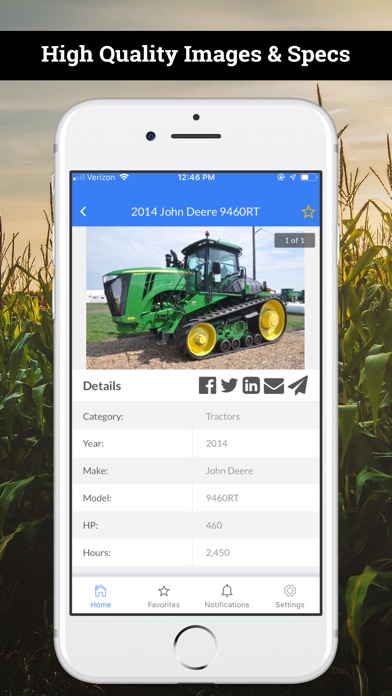In the image, a white cell phone is prominently displayed against the backdrop of a lush cornfield, with tall corn stalks and kernels visible extending throughout the background. The uppermost part of the picture is slightly overlaid by a semi-transparent rectangle containing the text "High Quality Images and Specs." The sky peeks through at the top of the frame, providing a hint of blue amidst the agricultural setting.

On the cell phone's screen, there is an image of a green tractor along with detailed information about it. The text reads "2014 John Deere 9460RT" and specifies various details such as the category: "Tractors," year: "2014," make: "John Deere," model: "9460RT," horsepower: "460 HP," and hours of use: "2450."

At the bottom of the phone's interface, several icons are visible, including a home button, a star for favorites, a notifications bell, and a settings gear. Additionally, there are social media links available for further interaction. Overall, this photo showcases technology and agriculture, highlighting the modern connectivity and detailed information accessible through mobile devices in an agricultural context.